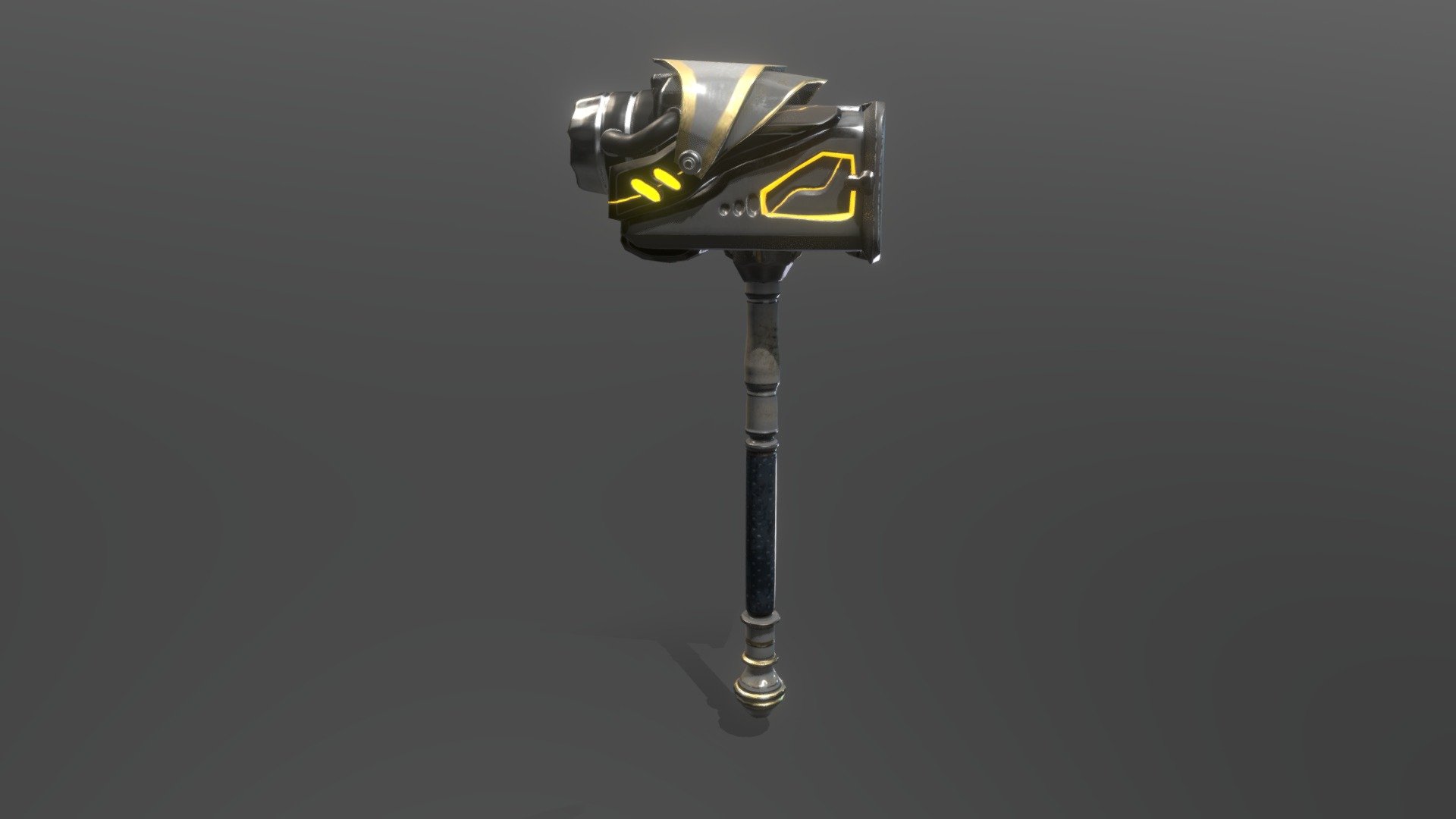The image is a detailed 3D rendering set against a completely solid dark charcoal background. Central to the scene is a peculiar object that appears to be a hybrid between a hammer and a staff, suggesting it could be a weapon or tool from a video game. The object features a long shaft with a hammerhead at the top, elaborately designed and not of a basic hammer nature. The hammerhead showcases ornate coverings in yellow and clear colors, with fluorescent yellow designs on its sides. Detailed scrutiny reveals a grey and gold visor-like element on the top, covering what seems to be a lens on the left side, and a latch mechanism resembling an American-styled postbox on the right. The dark grey equipment is composed of metal and plastic, with a cylindrical element at the back and a flat, square front. The shaft is wrapped with plastic rubber, tapering down to a knob at the bottom, casting a subtle shadow onto the grey background, enhancing the digital illustration’s depth and realism.